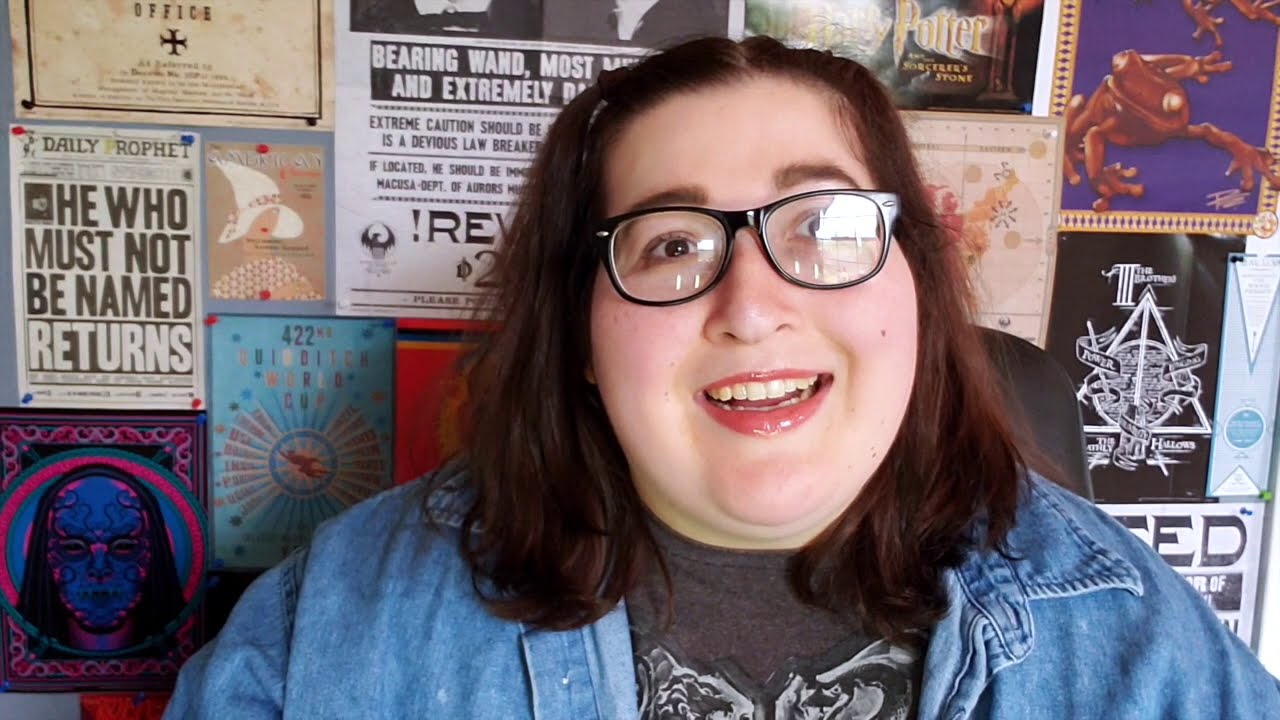The image showcases a large woman seated in an office chair, positioned centrally. She has shoulder-length brown hair with a reddish tint, parted to reveal her forehead. She wears thick black horn-rimmed glasses with a noticeable glare, and her bright red lipstick highlights her smile, revealing her teeth. Her eyebrows are quite bushy. She is dressed in a blue denim jacket over a black graphical t-shirt, which appears to have a light gray and black crest that is partially visible, possibly featuring a lion and a snake.

In the background, there is a collection of fandom posters, most notably from the Harry Potter series. Prominent among them is "The Daily Prophet" poster with the headline "He Who Must Not Be Named Returns." Other posters include various Harry Potter-themed graphics, such as a wanted sign and what appears to be the Harry Potter logo. Additional posters display varied colors, including blues, browns, whites, blacks, and some pinkish reds.

The overall setting suggests that the woman might be giving a speech or engaged in a conversation, as evidenced by her expression which shows her mid-sentence. The wall filled with vibrant, themed posters provides a colorful and engaging backdrop for the image.